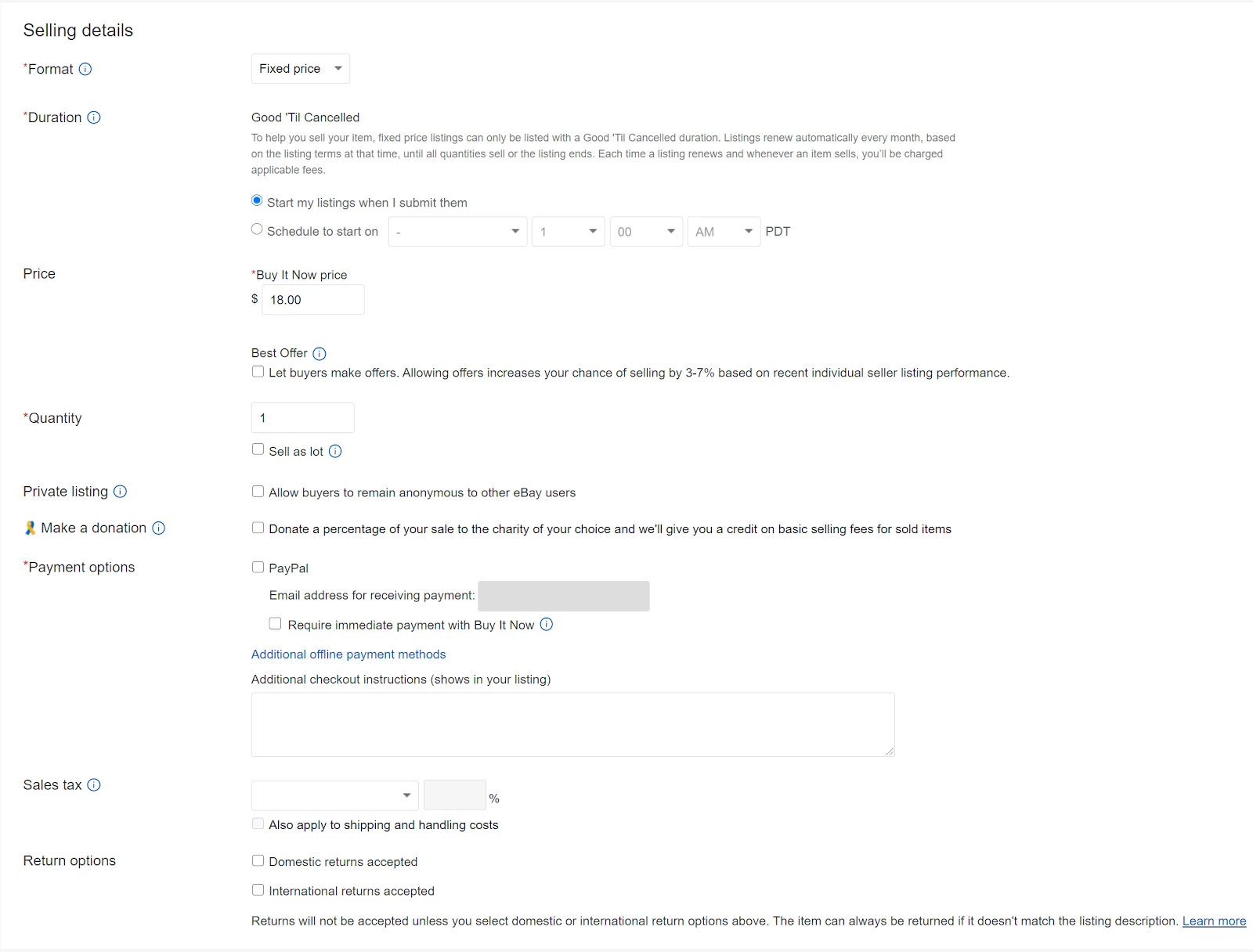A detailed screenshot of an eBay listing setup page. The screen displays various parameters for selling an item, and it's partially filled out with some default and user-defined values. Key details include:

- **Selling Details:** Information relevant to the item being sold.
- **Format:** The selling format is set to **Fixed Price**.
- **Duration:** The duration of the listing, though not fully visible.
- **Start Listings:** The option to "Start my listings when I submit them" is selected.
- **Schedule Listing:** Users have the option to schedule their listing instead of starting it immediately.
- **Buy It Now Price:** Set at $18, indicating the platform is indeed eBay.
- **Best Offer:** An option to let buyers make offers, with a note that allowing offers can increase the chance of selling by 3-7% based on recent seller performance.
- **Quantity:** Set to one.
- **Sell as a Lot:** A checkbox for selling items as a lot, which is not enabled in this screenshot.
- **Private Listing:** Option to allow the buyer to remain anonymous to other eBay users.
- **Make a Donation:** Sellers can choose to donate a percentage of their sale to a charity of their choice, with a note about receiving a credit on basic selling fees for sold items.
- **Payment Options:** Includes fields for a PayPal email address (left blank), an option to require immediate payment with Buy It Now (left blank), and additional offline payment methods (also left blank).
- **Sales Tax:** Indicates that sales tax is applicable, including shipping and handling costs.
- **Return Options:** Fields for return options are present but left blank.

The form appears to be in the process of being filled out, awaiting further input to complete the listing setup.